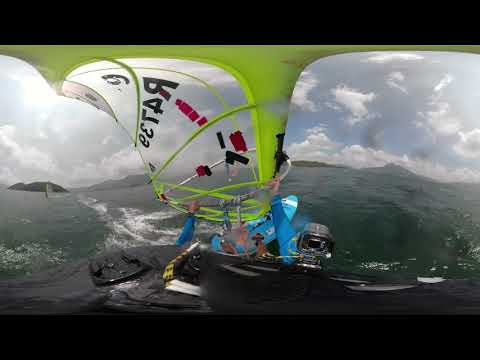The distorted, low-resolution image appears to be taken from an action camera, possibly mounted on someone's head or an object. It captures a vibrant boat equipped with a light green canopy and adorned with black lettering "R4736" and a number "9" prominently displayed on the left side. A striking blue surfboard with a white strip around its front tip is positioned at the back. The boat’s black engine, featuring some yellow lines, is centrally located. The water in the background is a blend of green and gray hues, featuring a white streak trailing behind the boat towards the left, indicating movement. In the scene, a person in a brown shirt and hat is visible, suggesting they might be operating the boat or windsurfing, as their arms and body are slightly visible. Surrounding the boat are choppy, high waves, hinting at a dynamic aquatic environment, possibly the ocean. In the distance, a dark-colored building and mountains provide a dramatic backdrop against a sky marked by faint blue tones mixed with prominent black and white strips.